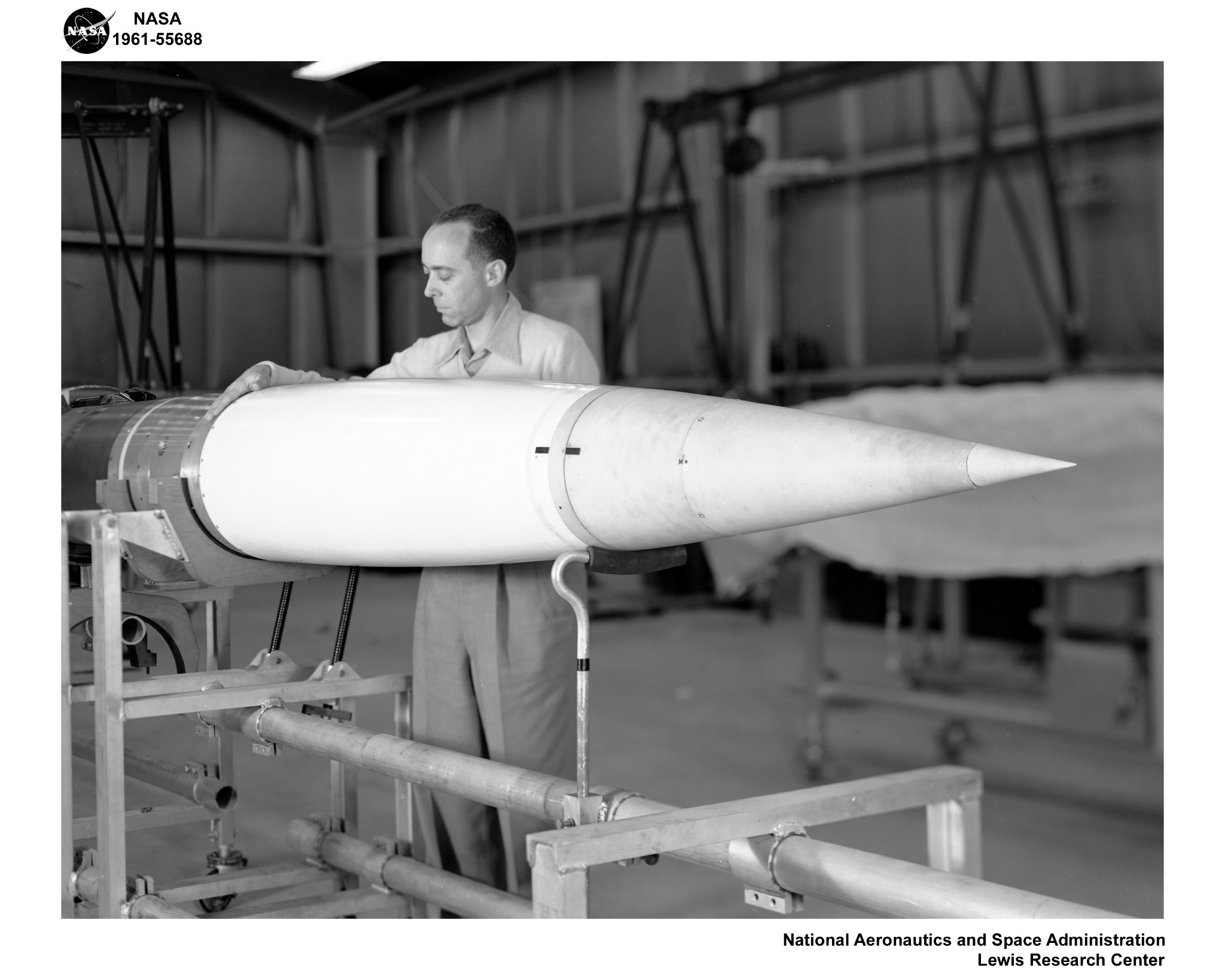This black and white photograph, titled "NASA 1961-55688" and marked with the NASA symbol, shows a man working on a pointed, conical missile, approximately 8 feet long. The missile, positioned horizontally on a metal holder with round pipes and square braces, features a white tip and a metallic base. The man, appearing to be in his 40s, has short, balding hair and wears loose trousers and a collared shirt layered with a 50s style top. The setting is an expansive warehouse or hangar with high ceilings and crane structures, likely depicting the Lewis Research Center of the National Aeronautics and Space Administration. His specific task remains unclear, but his hand placement suggests an inspection or construction activity related to the missile.